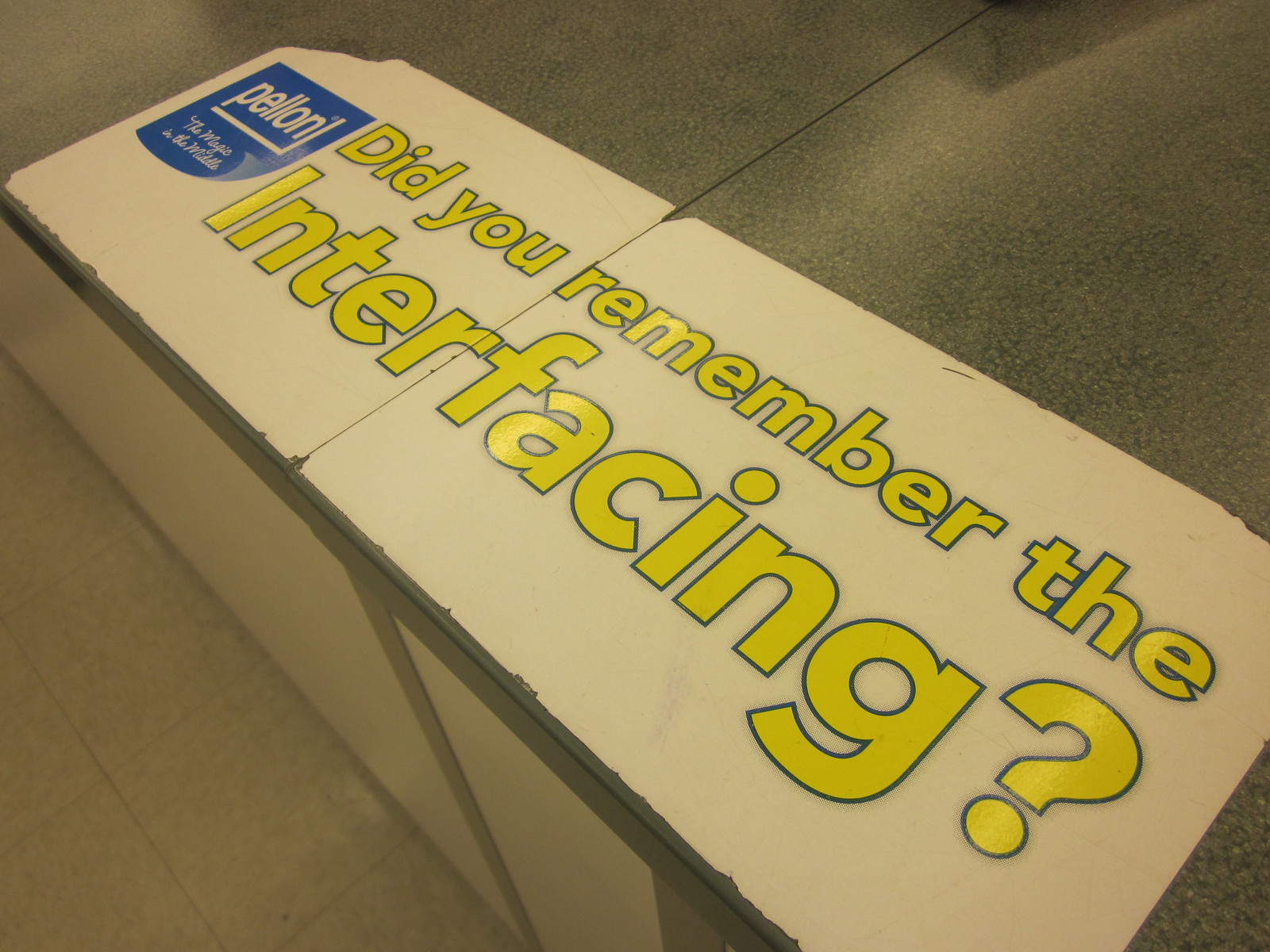The indoor photograph depicts a sign placed on a grey platform within what appears to be a warehouse setting. The platform, worn and chipped, supports a large rectangular block in white. Prominently displayed on this block is the phrase "Did you remember the interfacing?" written in yellow text bordered by blue, capturing immediate attention. On the top left corner of the sign, the word "P-E-L-L-O-N" is clearly visible in white lettering, accompanied by smaller, cursive text beneath it, though the latter is too unclear to decipher. The image, likely taken with an older digital camera or phone, exhibits signs of age and wear, both in the condition of the sign and the grimy, worn floor beneath. Despite the overall poor lighting and quality of the photograph, the details of the sign remain distinguishable, suggesting its importance or relevance in the depicted scene.